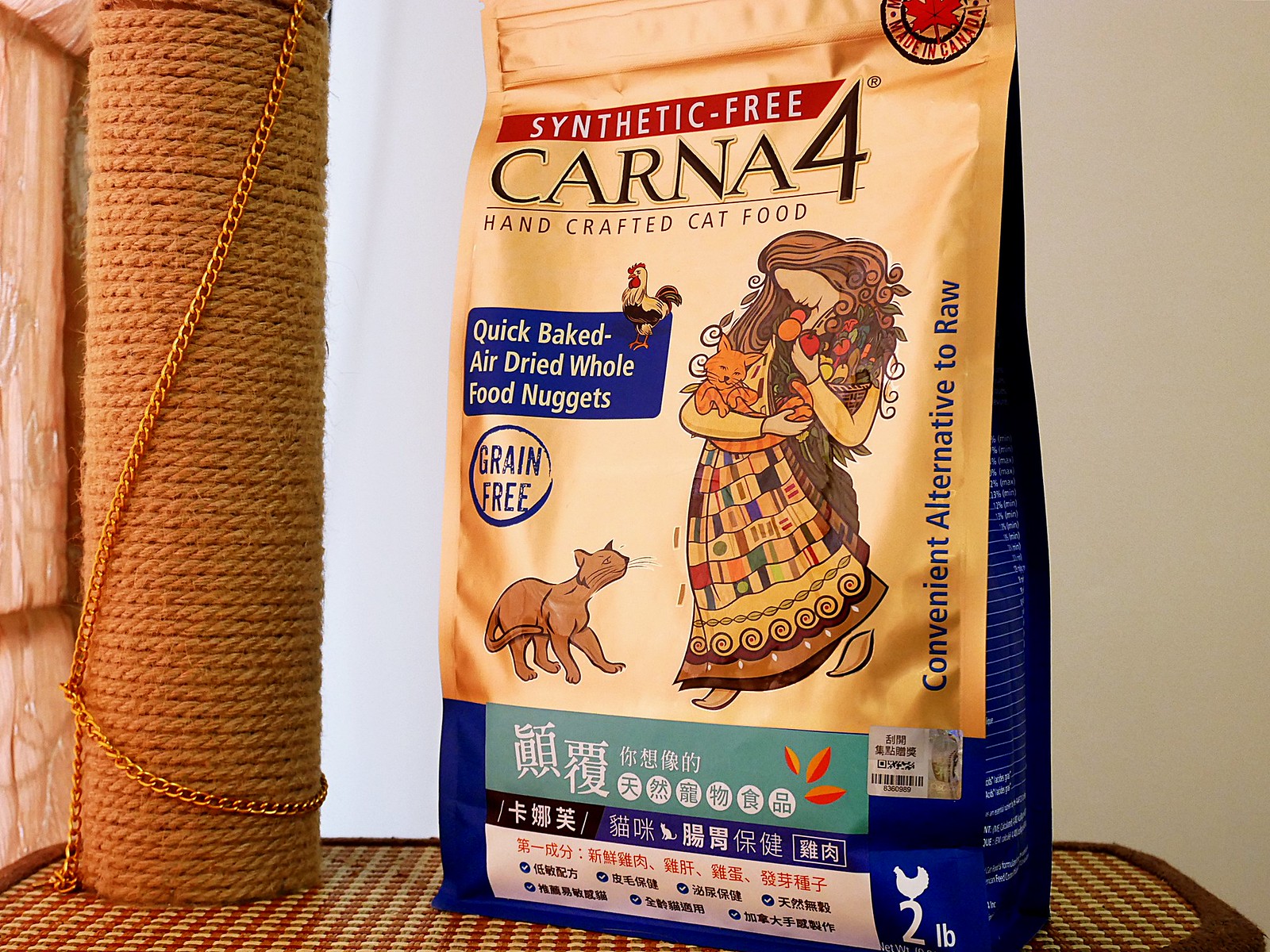The image depicts a vibrant bag of handcrafted, synthetic-free cat food prominently placed on a table with a wicker-like surface. The bag is a striking mix of blue and yellow, with bold white and black lettering that reads "Karna 4 Hand Practiced Cat Food" and "Quick Blended Air Dried Whole Food Nuggets." A small red line and a blue flag further highlight the distinguishing features of the product, such as "grain-free" and "convenient alternative to raw." The packaging includes a charming illustration: a woman in a vividly colored dress adorned with yellow, green, and blue squares, holding an orange cat and a bouquet of vegetables. Next to her, a smiling brown cat gazes up adoringly. A picture of a chicken hints at the product’s primary ingredient. Despite the presence of Chinese writing, a label confirms the food is made in Canada. The scene is set against a light grayish wall with a window draped in a white curtain, beside which stands a tall sisal rope cat scratching post with a metal chain wrapped around it. The overall setting suggests a cozy and well-loved space for feline companions.